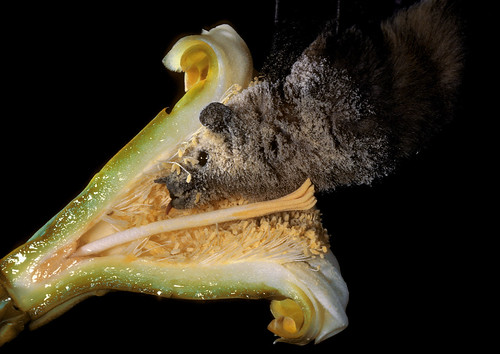This close-up digital photograph features a vividly detailed cross-section of a large, green flower with a jet black background. The flower’s outer edges are moist and gelatinous green, transitioning to a lighter, almost furry green shade as they approach the center. The center reveals an arrangement of white petals, some rolled at the edges, and intricate yellow pollen-covered structures, including smaller stems and a prominent large one. Dominating the upper portion of the image is a rodent-like creature, possibly a mouse, with a grayish-brown to almost black fur depending on the lighting. Its head is buried deep into the flower's central structures, blending into the scene with its distinctive black eye and ear visible amid the pollen-covered white interior. Two projections, appearing man-made, seem to hold the creature in place, enhancing the mysterious and intricate composition of the photograph.